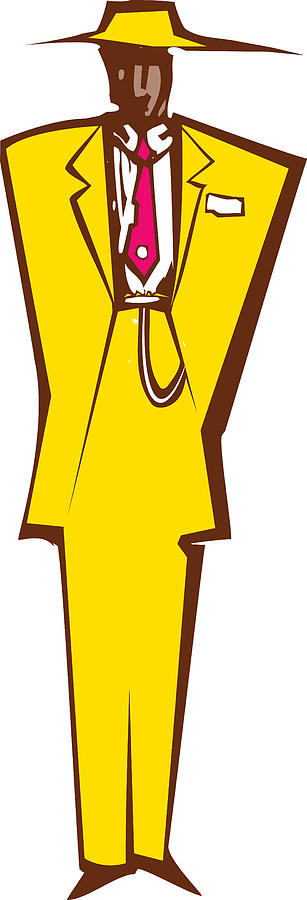This highly stylized illustration depicts a figure in a vibrant yellow suit, characterized by simple yet bold lines. The suit includes a broad yellow jacket with wide, pointed shoulders, yellow pants, and brown, triangular shoes. The figure wears a white collared shirt and a red tie adorned with a tie pin. A detail of the outfit suggests a pocket watch or chain looped around the belt. The face, rendered in dark and light brown shades, is minimally defined and appears to be turned to the right. The figure's angular hat, echoing the wide-shouldered style, features a wide brim that extends further on the right side compared to the left. The entire illustration carries an abstract, possibly Art Deco influence, with thin, angular, and pointed elements throughout, accentuating the figure's modernist aesthetic. The skin tone suggests the figure is African-American, adding further depth to the rich visual elements.